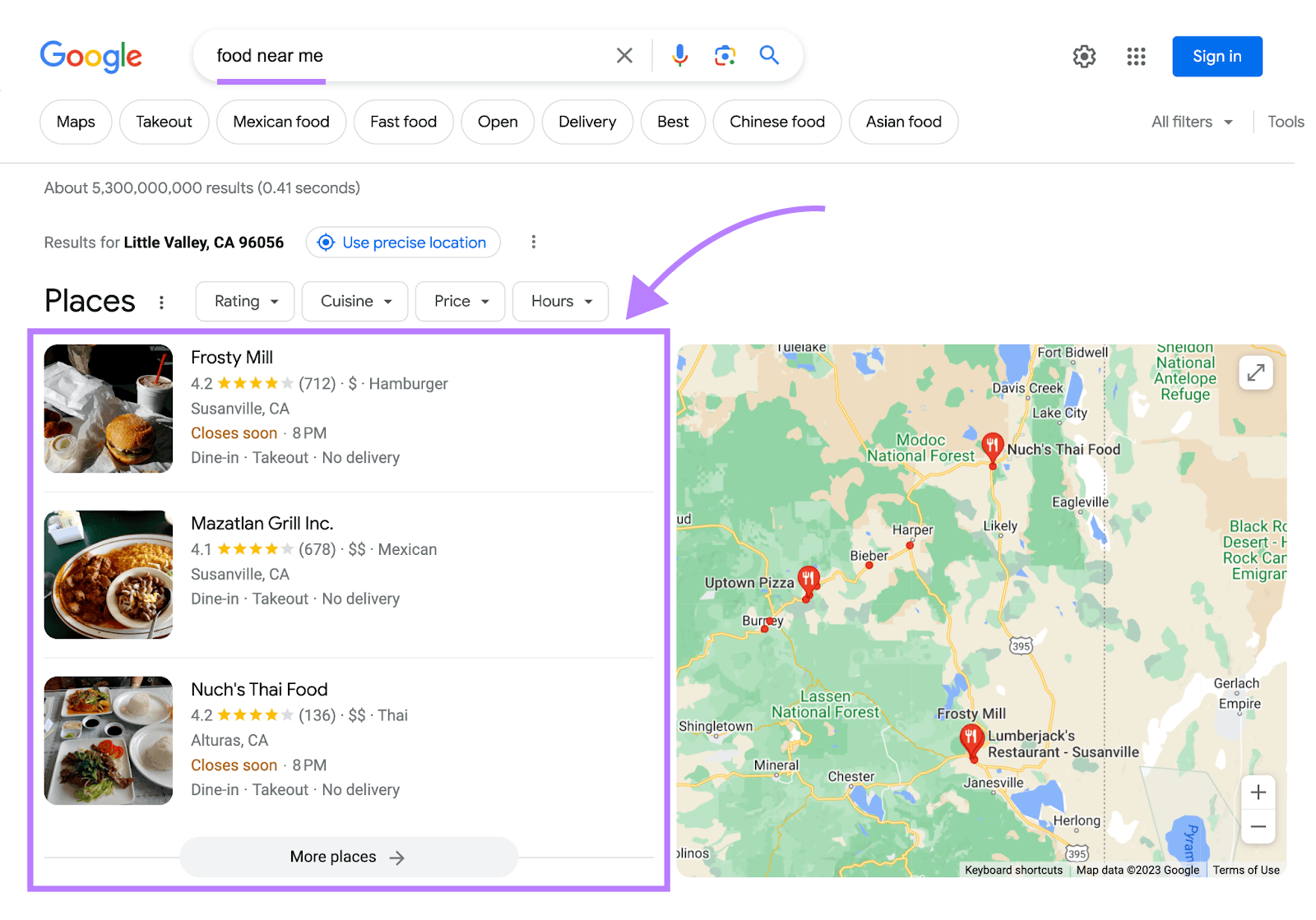A screenshot of a Google search page is displayed. At the top, the Google logo is prominently featured. Below it, a search query reads "food near me," underlined in purple. Adjacent are icons including an 'X' for clearing the search, a microphone for voice search, a camera for image search, a gears icon for settings, and a cluster of dots representing a menu. A blue "Sign In" button is evident, as well as a circular icon linking to Google Maps.

Categories like "Takeout," "Mexican food," "Fast food," "Open," "Delivery," "Bus," "Chinese food," "Asian food," "All filters," and "Tools" are visible. The search yields approximately 5.3 billion results in 0.41 seconds, localized for Little Valley, California, 96056, USA.

Key search results and their details are as follows:

1. **Frosting Mill** - Rated 4.2 stars, located in Susanville, California. Closes at 7 PM and offers takeout services.
2. **Monza Elan** - Appears on the list but with unclear additional details.
3. **Google Incorporated and Red Bull** - Mentioned without context.
4. **Thai Food, Alturas, California** - Rated 4.2 stars.
5. **Niche's Thai Food** and **Uptown Pizza** - Prominently visible on the right side of the search results.
6. **Lumberjacks Restaurant, Susanville** - Also included in the search results.

The screenshot captures various details such as places, ratings, cuisine types, price ranges, business hours, and additional related search information.